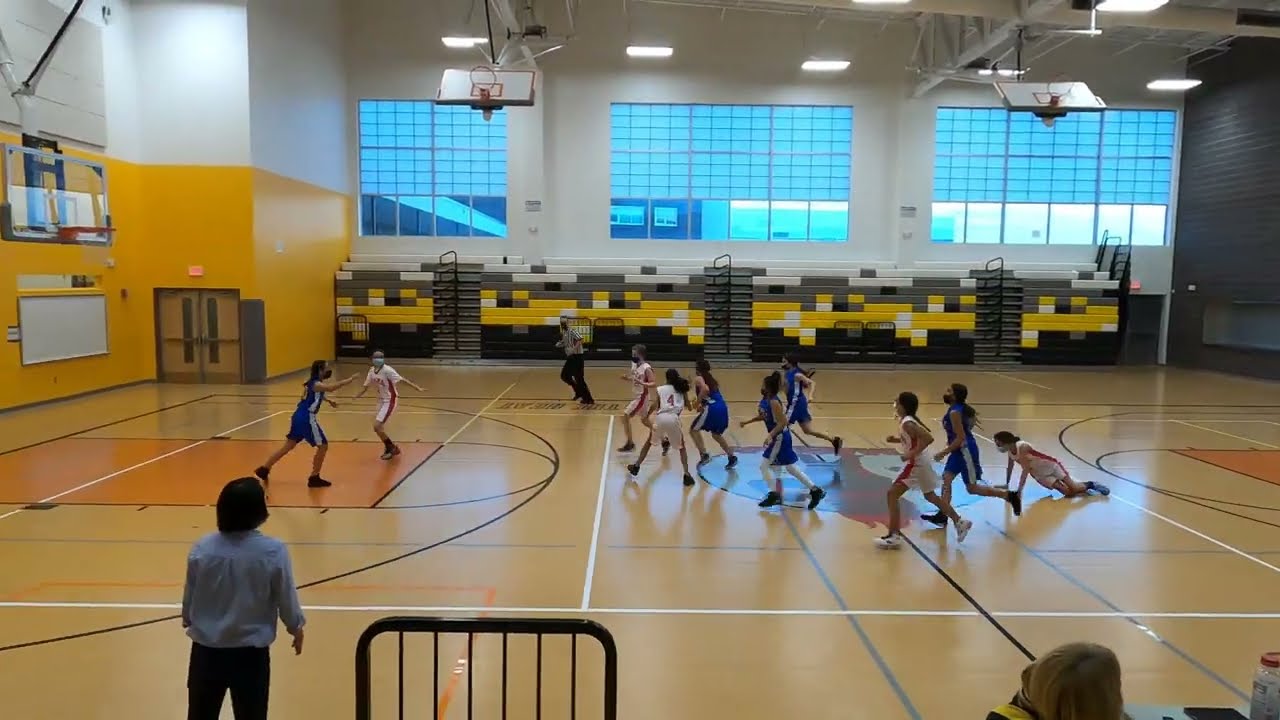In this horizontally aligned rectangular image, a high school girls' basketball game is captured in action within an indoor gym. The gym floor features a standard light brown wooden surface with black, white, and blue lines marking the court boundaries. Two teams are on the court: one in blue shorts and sleeveless jerseys, and the other in white shorts and sleeveless jerseys. A referee in black pants and a white and black striped shirt is running towards the players, trying to get a good view of the game. The players are actively engaged, with one player from the white team having fallen to the ground and about to get up, and the ball's location obscured by the players.

The far wall of the gym has bleachers that are currently unoccupied and pushed in. Just above the bleachers, large rectangular windows are embedded into the white-painted wall. The wall on the left side of the frame is painted yellow on the bottom half and white on the upper half. Visible in the lower right corner of the image is the head of a blond-haired individual, while in the lower left corner stands the coach in a long-sleeve shirt and black pants with short black hair. A single basketball goal is visible on the left, with the right side of the image cutting off before revealing the other goal. The bleachers behind the windows are gray, yellow, white, and black, reinforcing the vibrant setting of this lively basketball match.